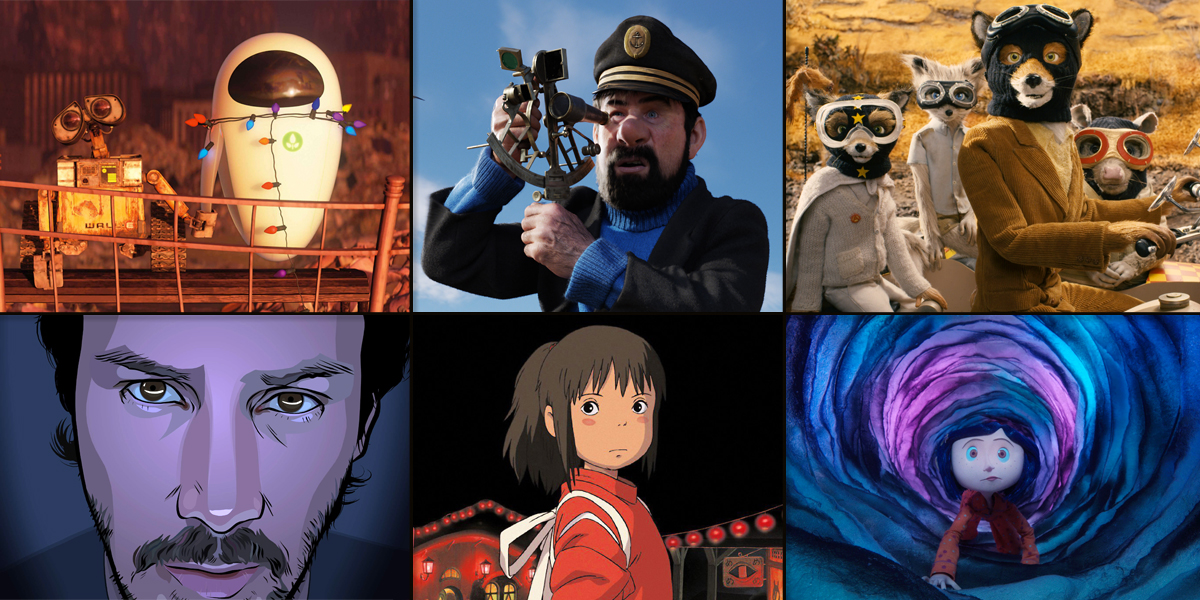The image presented is a horizontal rectangle composite of six distinct animated pictures arranged in two rows of three. 

- In the top row, the far-left picture showcases two robots standing on a bridge with a visible railing in front of them. The robot on the left has a square brown body and a short neck with two prominent eyes as a head, while the robot on the right is white, egg-shaped with a black screen at the top, and is holding hands with the first robot. 

- The top middle picture features an older man in sailor clothing, including a black jacket, a blue sweater, and a sailor's cap adorned with gold lines and an insignia. He is holding an instrument resembling a protractor in his hands.

- The top right picture depicts a group of animals on motorcycles, all wearing goggles. The group includes a fox at the front, a pig to its right, another fox or fox-like animal behind, and possibly a cat completing the group.

- In the bottom row, the picture on the left is a close-up of a cartoon man's face with a mustache, some beard growth, and black hair on the sides. His face is cut off at the forehead.

- The bottom middle image captures a cartoon little girl with brown hair and bangs, facing right but looking back over her shoulder. She is depicted against a background with strung lights, hinting at a festive or fair setting.

- The bottom right picture shows another little girl with shoulder-length dark hair, wearing something orange, crawling through a blue and purple tunnel that features swirling patterns on the sides.

The collection appears to be a montage of various animated works, each offering a unique visual and thematic element.